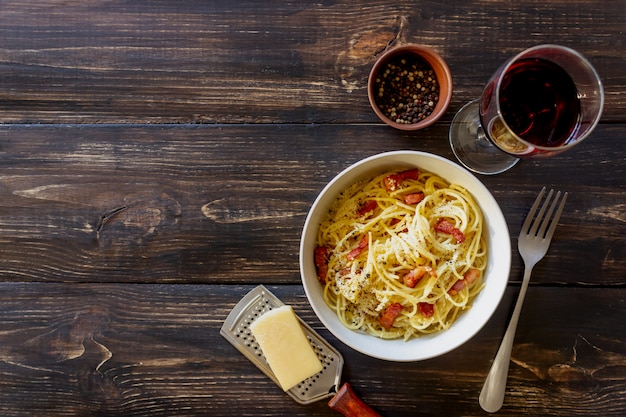A beautifully rustic meal is captured from an overhead perspective, set on a wooden table with charming, natural imperfections. The table's surface showcases a mix of dark and light brown hues, punctuated by knots that add character and warmth to the scene. On the right side, a vibrant array of dining elements is artfully arranged. An orange or reddish cup sits with a mix of black and light brown seeds, adding a touch of earthy texture. Next to it, a sophisticated wine glass holds deep red wine, ready for savoring. A gleaming silver fork lies poised for use, while a cheese grater with a wooden handle and a delectable piece of white cheese promise a delightful finishing touch. The centerpiece is a pristine white bowl filled with creamy pasta, speckled with vivid red tomato pieces and a dusting of what appears to be freshly cracked black pepper, adding a flavorful contrast. The entire composition is a feast for the eyes, inviting and tantalizing, perfectly framed by the bird's-eye view.